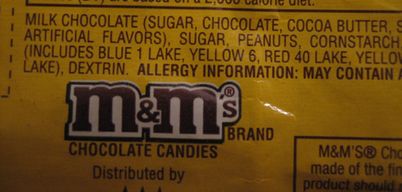A package of Peanut M&M's is prominently displayed, recognizable by its vibrant yellow color characteristic of the brand. The packaging shows the M&M’s brand chocolate candies logo and features a partial ingredients list, which includes peanuts and milk chocolate. A detailed but incomplete list of ingredients is visible, listing components such as sugar, milk chocolate, chocolate, and cocoa butter, followed by artificial flavors. Some of the text is cut off, disrupting the flow of information. The visible text resumes with additional ingredients: sugar, peanuts, corn starch, and an assortment of food colorings that include Blue 1 Lake, Yellow 6, and Red 40 Lake. However, some words remain partially obscured, showing only fragments like "yellow…lake." The label also contains partial allergen information, which is assumed to warn about the presence of peanuts or other nuts.